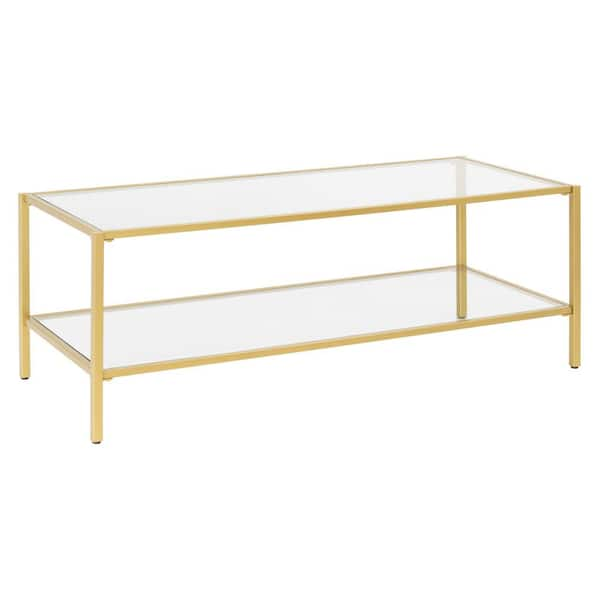In this photo, we see a rectangular coffee table set against a stark white background. The table features a sleek, minimalistic design with a combination of materials and colors. Its top and bottom surfaces are made of clear glass panes, allowing visibility through both levels. The legs and frame of the table are constructed from a material that appears to be wood—or possibly plastic—finished in a light yellow or brown color, depending on the lighting. Each of the four legs is equipped with small black stoppers or screw-on feet that elevate it slightly off the ground and provide stability. The table is devoid of any items, making its modern and simplistic aesthetics stand out.